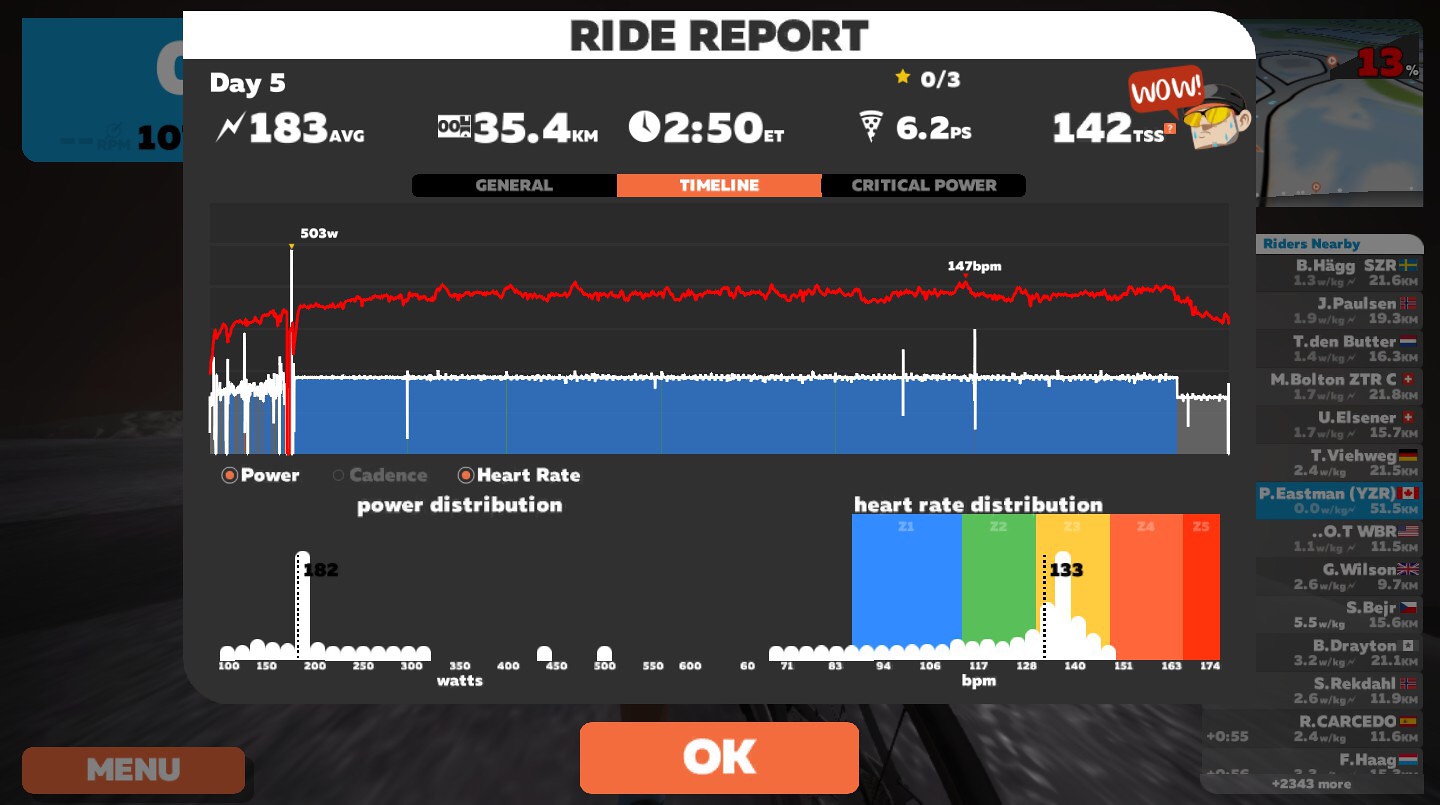This image depicts a detailed screen from a video game or fitness app showing a Ride Report. At the top in a white bar with black text, it prominently reads "Ride Report." Below that, the centerpiece of the screen is a black rectangular pop-up displaying various metrics: "Day Five," "183 average," "35.4 kilometers," "2.50 Eastern time," "6.2 PS," and "1.42 TSS." Centrally located, there is a graph featuring a red squiggly line that illustrates heart rate distribution over the ride, with specific values indicating 133 as the average heart rate, and a range spanning from 70 to 174. The graph is overlaid on a blue bar beneath the red line. The bottom corners of the image include interactive elements: an orange rectangle reading "OK" on the right, and a slightly darker rectangle reading "Menu" on the left. Additionally, three tabs are visible at the bottom of the pop-up: "General" in gray, "Timeline" in white on an orange background, and "Critical Power" in gray. In the background, particularly in the top right corner, there's a map highlighting a 13% grade, contributing further details to the ride's context. Various user data from different countries indicate a global participation element in the app.